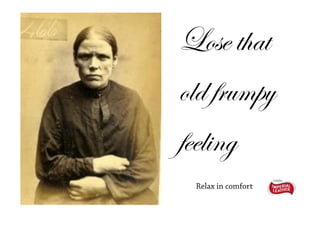The image appears to be a very dated black and white advertisement from the 19th century, possibly from the 1800s, characterized by its yellowish-gray, old-fashioned patina. The focal point of the advertisement is a solitary woman with a pale complexion, dark hair slicked back, possibly into a bun. She is dressed in a long-sleeved, buttoned-up black dress. The woman exhibits a stern or unhappy expression, suggestive of discomfort or annoyance, as she holds herself with crossed arms. Her demeanor might evoke a sense of hardship or weariness, reminiscent of personas from the Great Depression era despite the 19th-century attire.

On the right side of the image, there is cursive script that reads, "lose that old frumpy feeling." Directly beneath this, in regular text, are the words, "relax and comfort." Adjacent to this text is a small red logo, though the specific lettering is indecipherable due to its diminutive size. Additionally, the photo includes the number "466" in the upper left corner, further emphasizing its vintage nature.